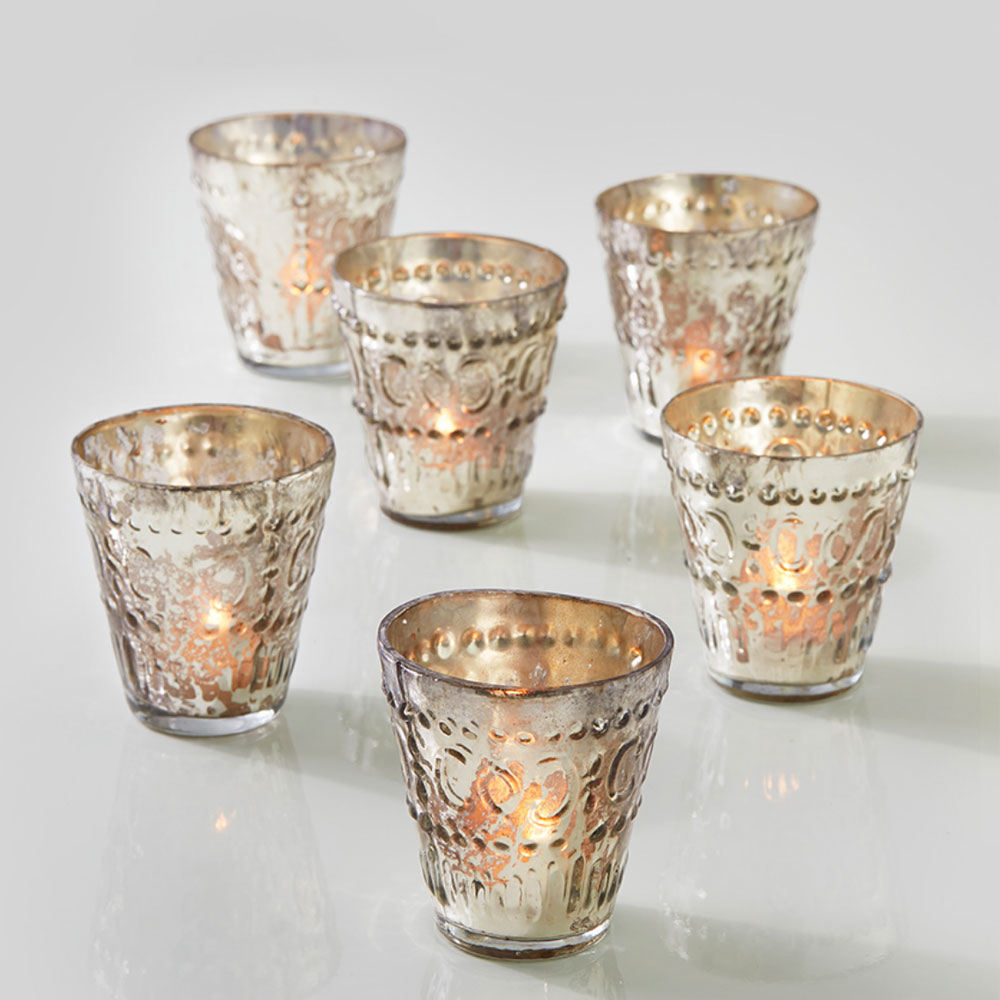In the image, there are six rustic-looking candle holders made of textured glass with a reflective metal coating inside, providing a blend of transparency and reflectivity. The glass has splotches where the coating is absent, allowing glimpses of the flickering flames within. The candle holders are characterized by rings of circles and squiggling lines that create a semi-circular design pattern on their outer surface. They are arranged on a glossy white table in an almost triangular formation, three in the front and three in the back, with the farthest one on the left set slightly further back. The candle holders also feature gold and white faded accents with divots and imprinted designs, although the specific letters or designs are unreadable. The glossy surface of the table reflects the candle holders, enhancing the rustic and glowing ambiance of the scene.